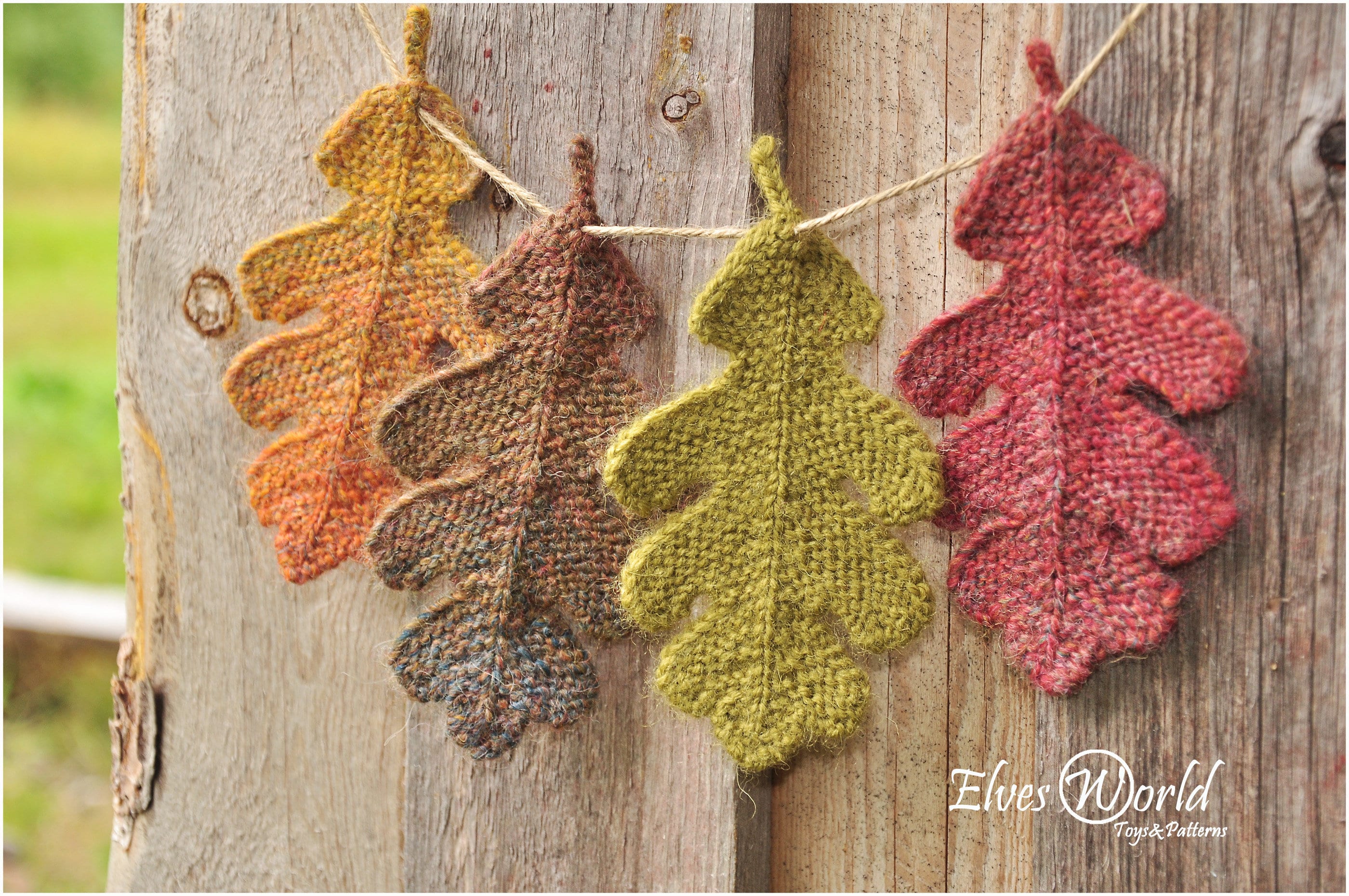This full-color, square photograph, taken outdoors during daytime under natural light, captures a serene scene. On the left side, the image features an open, green field, slightly blurred to emphasize the main subject. Dominating the center is a tan, smooth-faced wooden fence, bearing a couple of nails and knots, adorned with a piece of brown twine. Strung across this twine are four carefully crafted, crocheted leaves in a charming spectrum of autumnal colors: orange, brown, green, and red. Each leaf features a triangular top with two sets of symmetrical leaves branching out on either side, and a small stem at the top threading through the twine. In the lower right-hand corner, white text displays the company name “Elves World,” with “World” encircled, followed by “Toys and Patterns” in a distinct, playful font.